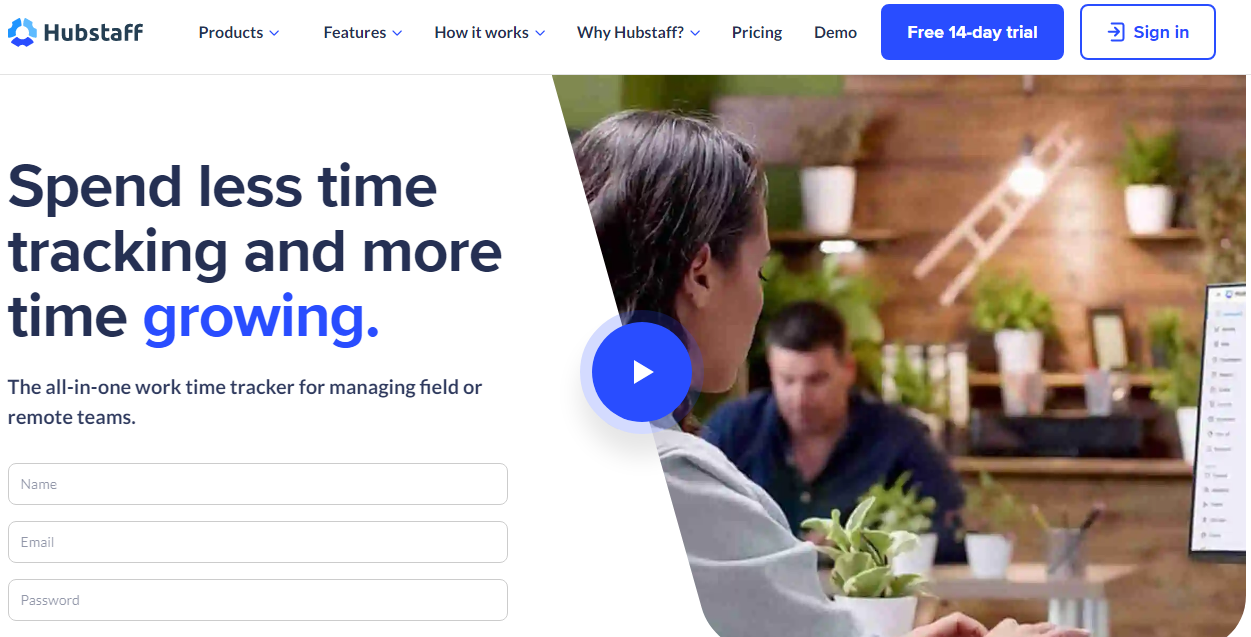The upper portion of the image features a white background on the left-hand side with a recycle logo in shades of blue and black, accompanied by the text "Hubstaff." On the right, there are several clickable buttons labeled "Products," "Features," "How It Works," "Why Hubstaff," "Pricing," "Demo." Below this, a blue banner with white text reads "14-day," and a white button with blue text says "Sign in," surrounded by a blue border. 

Beneath this, on the left-hand side, bold black text states "Spend less time tracking and more time," with the word "growing" highlighted in blue. Underneath, smaller black text reads, "The all-in-one work time tracker for managing field or remote teams." There is an input field section where users can enter their name, email, and password. In the center, a prominent blue circle with a white arrow pointing to the right acts as a play button.

The lower portion of the image showcases a stock photo of a man and a woman in a cozy, artsy plant shop. The woman, looking away from the camera, and the man, whose face is turned towards the camera but looking down, are surrounded by an array of plants and small white cups. The background features a beautifully crafted wooden wall with hanging plants and a suspended light, adding to the shop's artistic atmosphere. On the right-hand side, the woman seems to be looking at a computer screen or whiteboard, displaying what appears to be an email client or messaging interface.